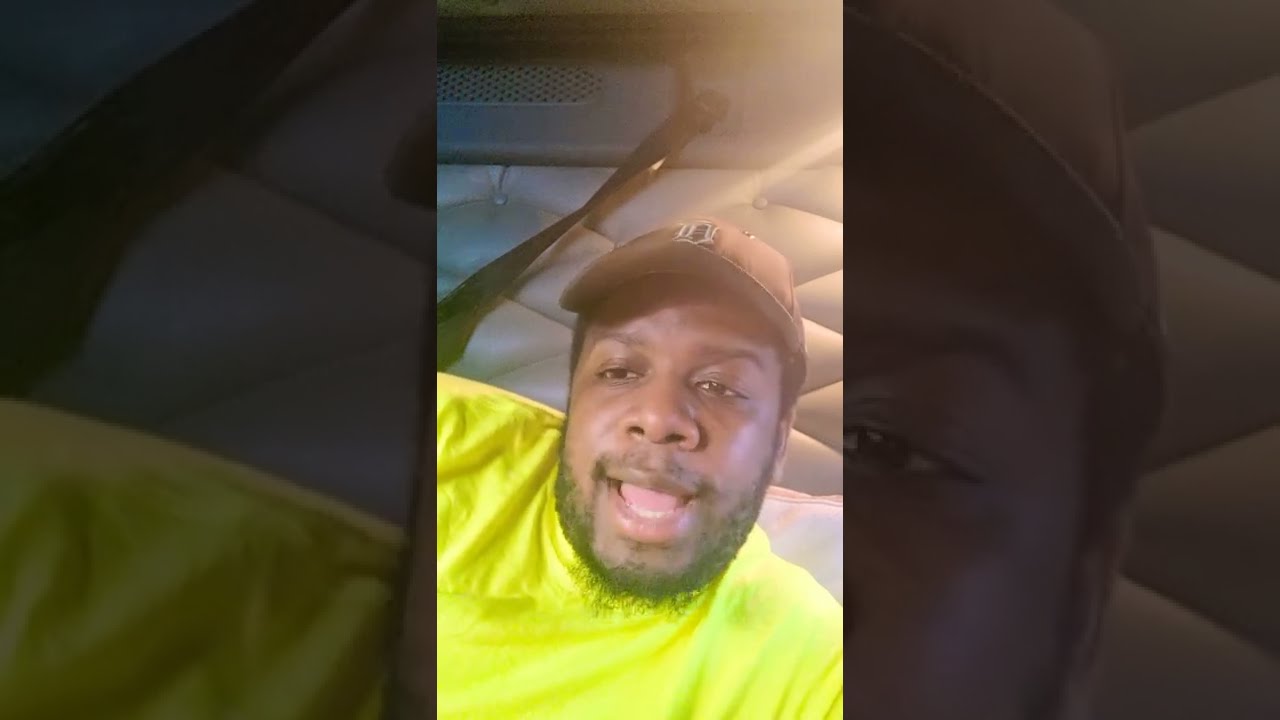The image captures an African-American man, prominently featured against the background. He is sporting a bright yellow shirt and a brown baseball cap. The man has a scraggly beard and a thin mustache over his upper lip. He appears animated and engaged in conversation, possibly recorded for a social media video on platforms like Facebook, TikTok, or Instagram, given the smartphone aspect ratio. The setting resembles an upholstered interior, likely of a vehicle like a bus, airplane, or perhaps a transport truck, inferred from visible details like a seatbelt strap and vent above the headrest. Light streams from the upper right, casting a glare that highlights his shirt. The backdrop is an enlarged, close-up section of the same image, further drawing attention to his animated expression and setting.